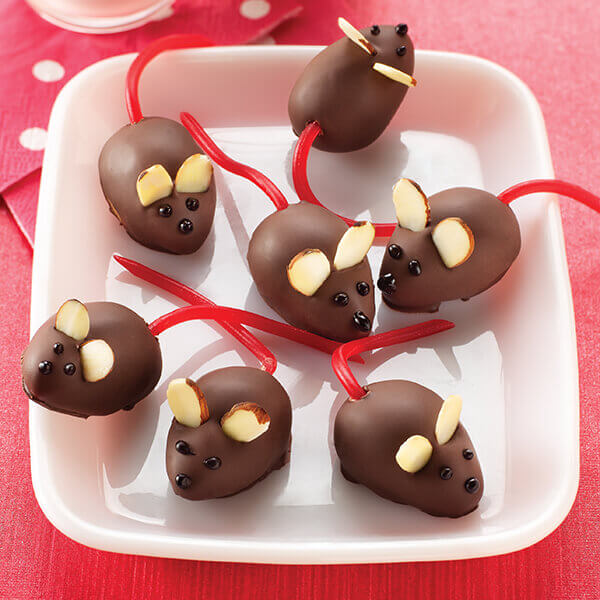In the center of the image, a square white plate rests on a red wooden surface. On this plate are seven chocolate mice, each adorned with almond slice ears, black eyes, and red Twizzler tails. Six mice form a cluster in the center, with three appearing to face the camera and the others positioned in various directions. A single mouse at the back faces upwards to the right. A red napkin with white polka dots is positioned at the top left corner beneath a partially visible glass cup. This whimsical arrangement suggests a festive setting, possibly a child's birthday party, making the mice look both adorable and delectable.